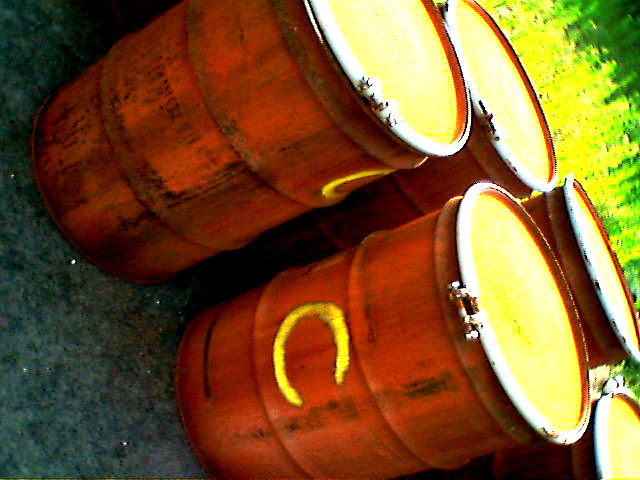The image, set outdoors, features five rusty barrels positioned at various angles atop a grayish-brown dirt surface. The barrels, which are a grungy, burgundy-brown color with a weathered appearance, have tops adorned with a white rim and a yellow center. Some of the barrels have letters painted in yellow, with one prominently displaying the letter 'C.' In the background, a gradient of green hues fills the scene, transitioning from a dark green at the top right to a bright yellowy-green toward the middle. The barrels are arranged with two in the front, two in the back, and the fifth partially visible at the bottom right. The background also features an array of grass and tall plants in different shades of green, adding depth and contrast to the image.